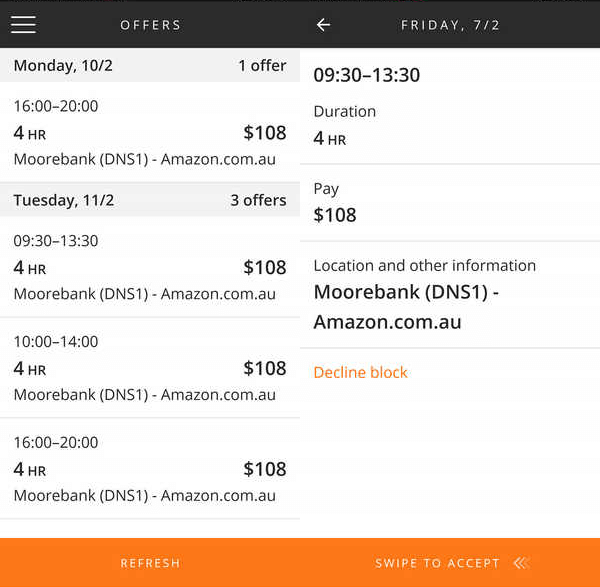The image depicts a job offering portal for Amazon, possibly tailored for the Australian market. It features several shift opportunities at a location referred to as "Morebank DNS1 Amazon.com.au." Each listing specifies a 4-hour shift with a consistent pay rate of $108. 

- The first job offer shows a shift time from 16:00 to 20:00.
- Another offer is from 11:00 to 15:00 on Tuesday.
- All job offers mentioned have a uniform duration of 4 hours and the same pay rate.

Users can refresh the listings and swipe to accept the job offers. The portal appears to be a streamlined interface for users to browse and accept job shifts efficiently.